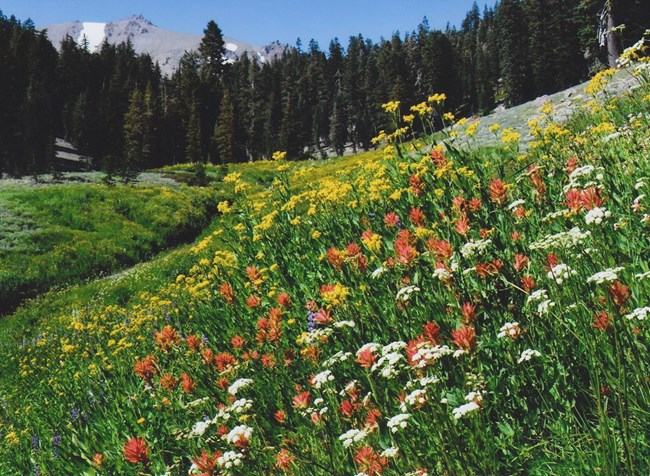The image showcases a stunning, lush meadow filled with a vibrant array of wildflowers, including yellow, red, pink, purple, blue, and white blooms set against a backdrop of tall, rich green grasses. The meadow is situated on a gently rolling hillside, speckled with clusters of flowers and dotted with charming rocks. A small, meandering brook runs along the left side, lined with similar colorful flora. The scene is framed by dense, towering evergreen trees, which extend diagonally from the left to the right, following the contours of the hillside. In the distance, a majestic, snow-capped mountain rises against a bright blue sky, adding to the picturesque beauty of the landscape. The vivid colors and natural elements evoke a serene, inviting atmosphere, perfect for a tranquil walk through nature.